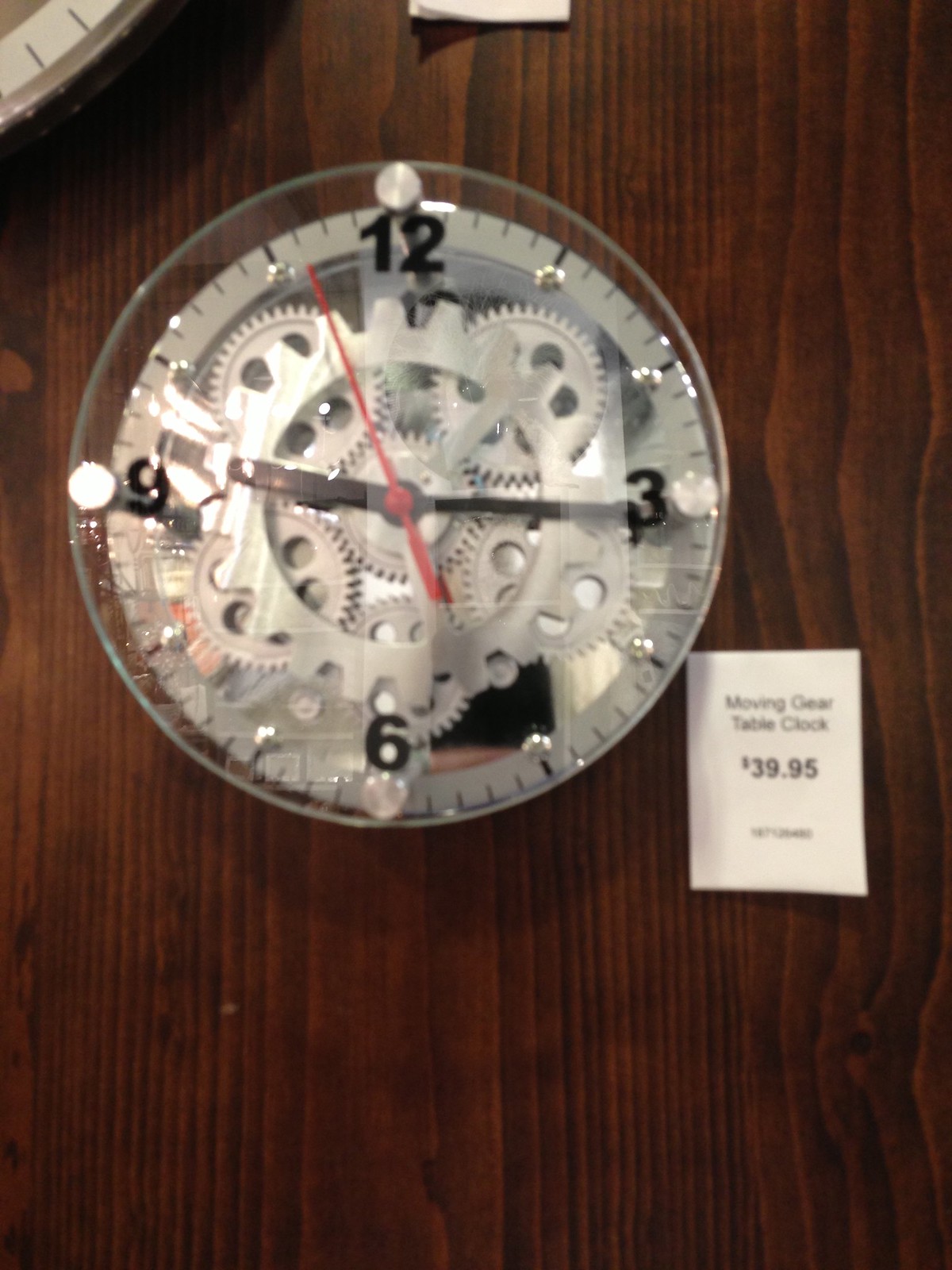The photograph showcases a transparent table clock sitting on a dark red wooden table. The clock face, made of clear glass, reveals a intricate array of gears inside. Four chrome pillars support the clock face, which features black hour and minute hands, and a red second hand. The face is marked with black numbers at 12, 3, 6, and 9 o'clock positions, and five-minute intervals are delineated with dots between each hour marker. A white paper sign to the bottom right of the clock reads "Moving Gear Table Clock, $39.95." The time displayed on the clock is 9:15.